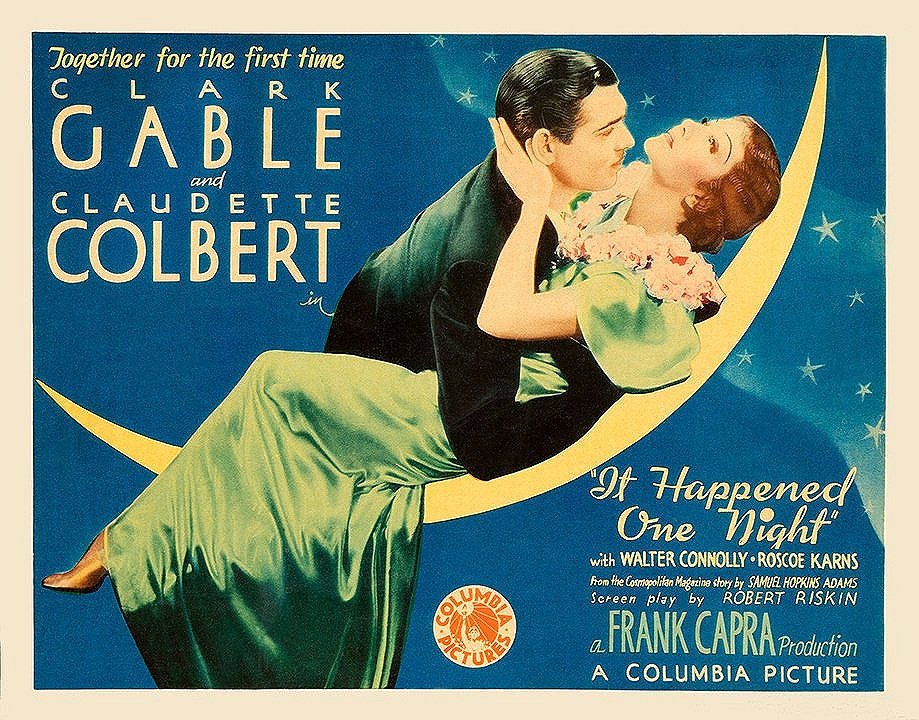This image is an old movie poster with a navy blue background featuring a crescent moon that appears to double as a hammock. The moon is yellow and stretches from the middle left-hand side to the upper right-hand corner. There is a streak of white stars resembling a galaxy running diagonally from the right-hand side towards the center. 

Lying on the moon, a woman in a shiny gray-green silk dress and adorned with a pink flower wreath tilts her head back, displaying her wavy brown hair. She is in an intimate pose, being embraced by a man with slick black hair, wearing a black suit.

In large white letters on the upper left, the poster announces, "Together for the first time, Clark Gable and Claudette Colbert." At the bottom, it reads, "It Happened One Night" with additional names "Walter Connolly, Roscoe Karns," and notes "A Frank Capra Production, a Columbia Picture." The image is horizontally oriented and rectangular in shape, capturing the enchanting essence of this classic film advertisement.